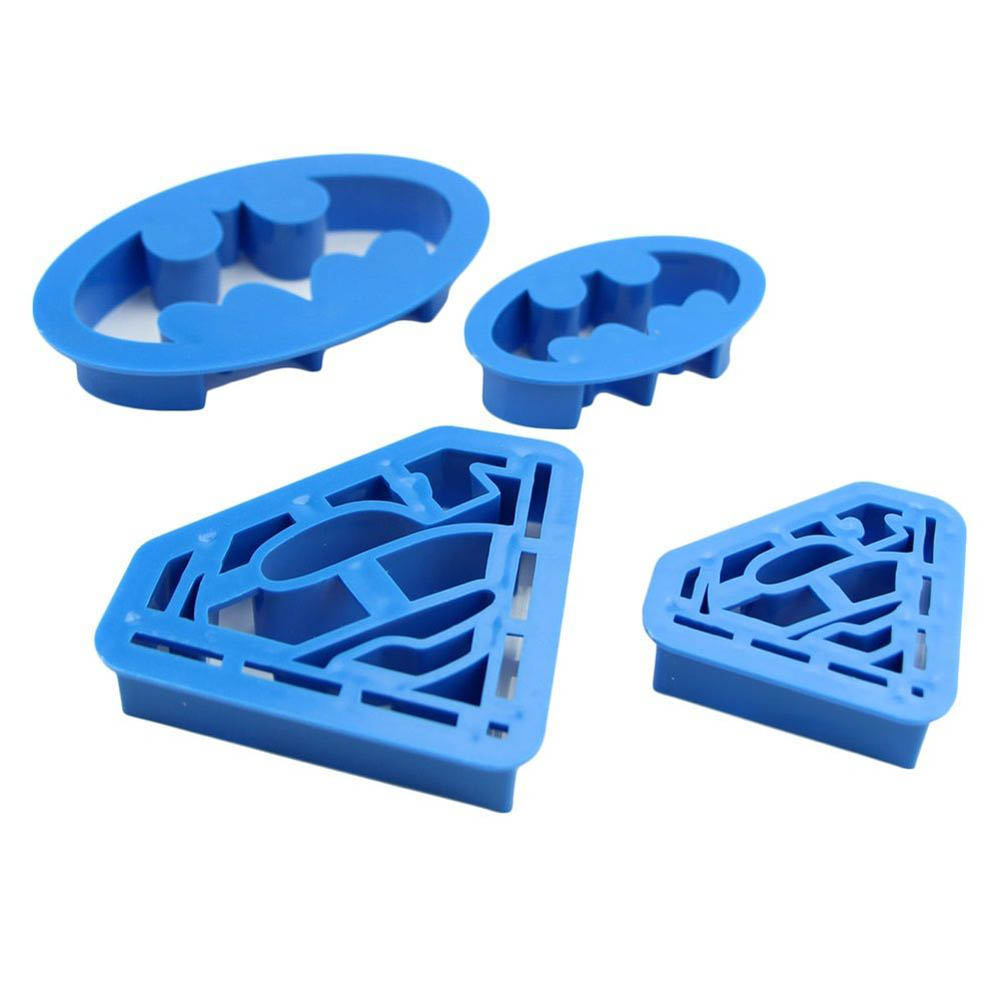The image showcases a set of light blue rubber or plastic molds designed for creating emblems of Batman and Superman, positioned diagonally on a solid white background as seen from a top-down angle. At the top of the image, there are two Batman molds, both featuring an oval shape with an outlined bat symbol. The left mold is slightly larger with a noticeable rim around the top that narrows towards the bottom, and is transparent enough to see the white beneath it. Its counterpart to the right is identical in design but smaller in size. Below these, two Superman molds are visible, each with a diamond shape housing the iconic 'S' insignia. Similar to the Batman molds, the Superman molds differ in size with the left one being larger. Both molds feature sharp edges to facilitate cutting through materials like clay or play-doh, and have no text or words imprinted. The overall composition emphasizes the detailed craftsmanship of these molds, highlighting their utility and aesthetic appeal.